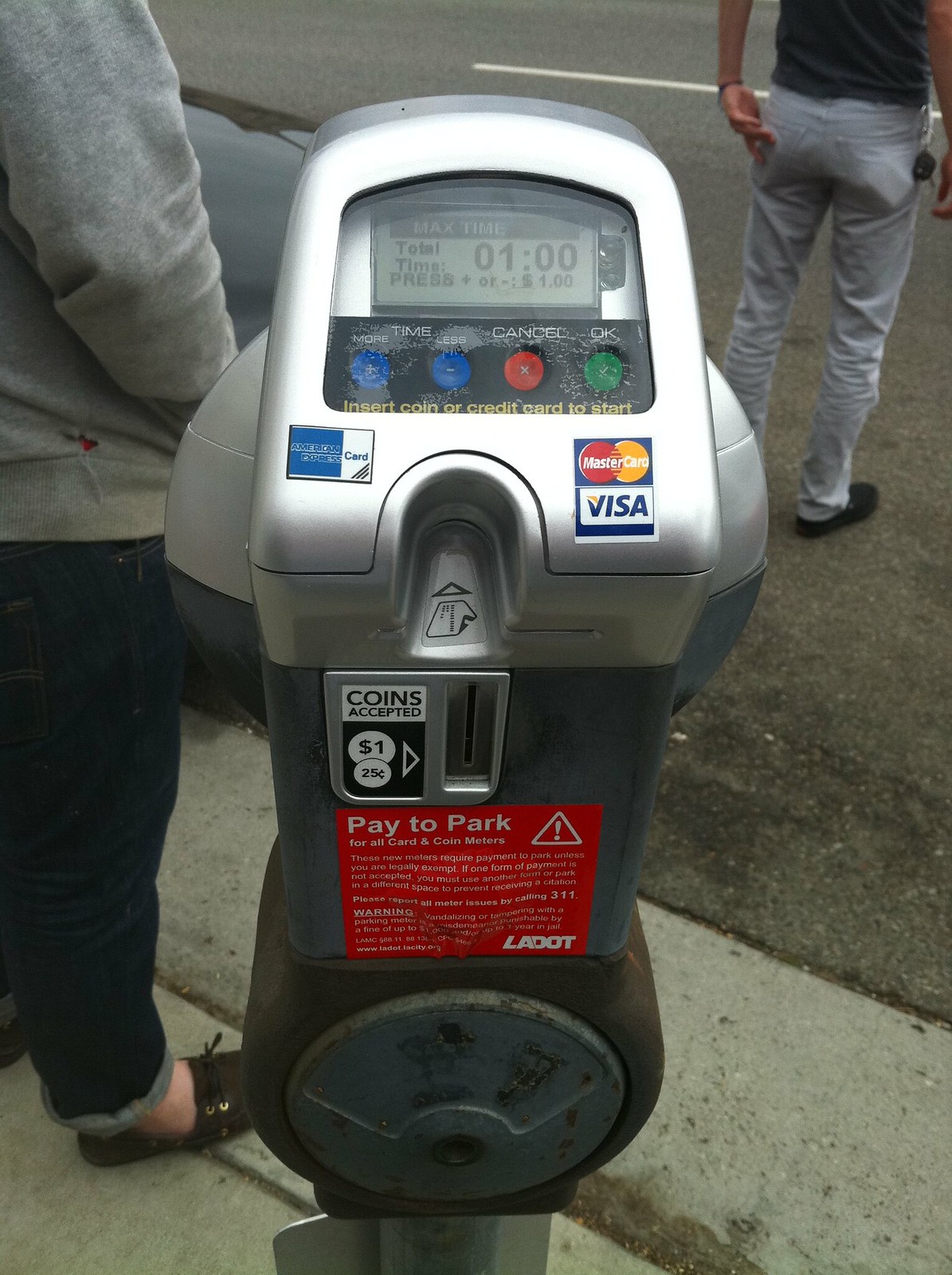This photograph, a close-up in portrait mode, captures a modern, somewhat weathered parking meter in detailed clarity, situated on a street during daytime. The meter prominently features a digital screen displaying "Max Time," "Total Time Pressed," a countdown timer, and a balance. Below the screen are four buttons: the first on the left is labeled "More Time," the second "Less Time," the third is a red "Cancel" button with an X in the middle, and the fourth a green "OK" button with a checkmark. The meter instructs users to "Insert Coin or Credit Card to Start," and it has a coin slot labeled "$1.25" adjacent to a label indicating it accepts MasterCard, Visa, and American Express cards. Above the coin slot is a credit card slot, and there is a red "Pay to Park" label under the coin slot. The top part of the meter is silver, with visible rust particularly noticeable at the bottom. In the background, part of a street and a black car are visible, as well as two people: a woman in jeans and a gray sweater standing to the left, and a man in skinny jeans and a black shirt a few steps ahead of her. The photo highlights the utilitarian features of the parking meter while showing a glimpse of the surrounding urban environment.